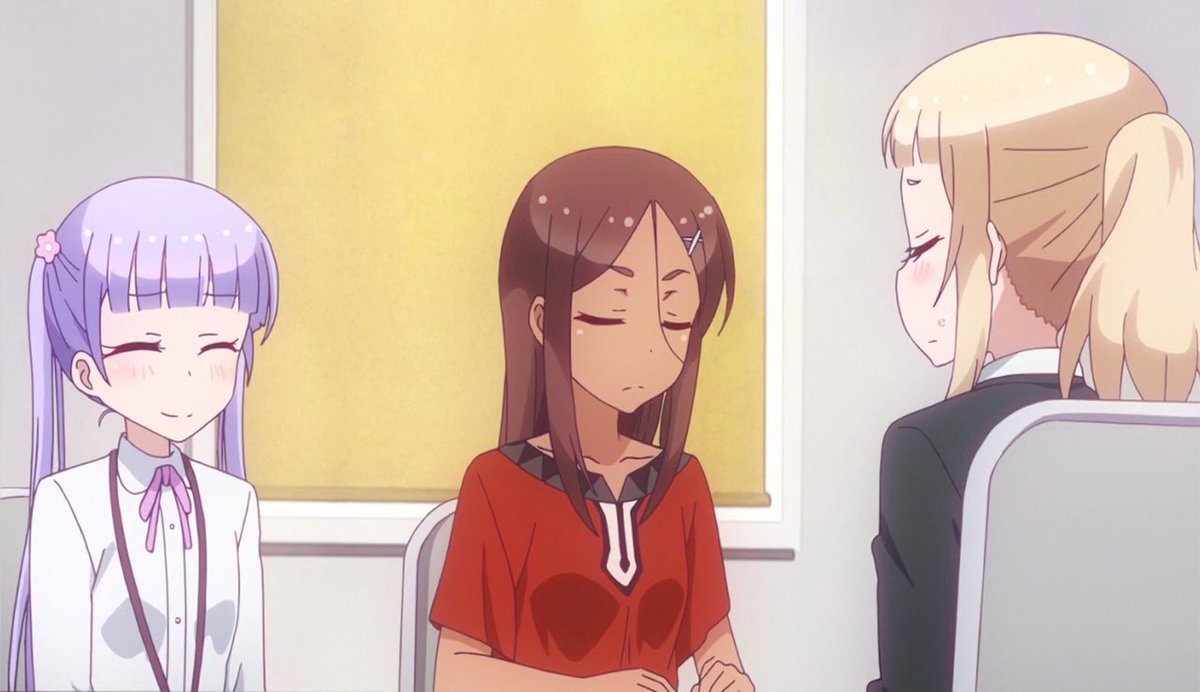The image depicts a vibrant, anime-style scene featuring three seated female characters against a background of a closed window with tan roman shades and a plain back wall. The character on the left, with pale skin and light lavender hair styled in pigtails with fringe bangs, adorns a small pink floral barrette. She is dressed in a long-sleeved white top accentuated with a pink bow and a reddish-brown chain. The central character with caramel-colored skin has loose brown hair held by a white pin, wearing a short-sleeved red top with a grey and black geometric border and a distinct white-bordered keyhole opening at the chest. The character on the right possesses golden blonde hair tied in a ponytail with fringe bangs, and she is dressed in a dark-colored jacket over a white top. All three characters have their eyes closed, evoking a serene atmosphere. The overall composition suggests a scene from an anime show or a manga comic book.